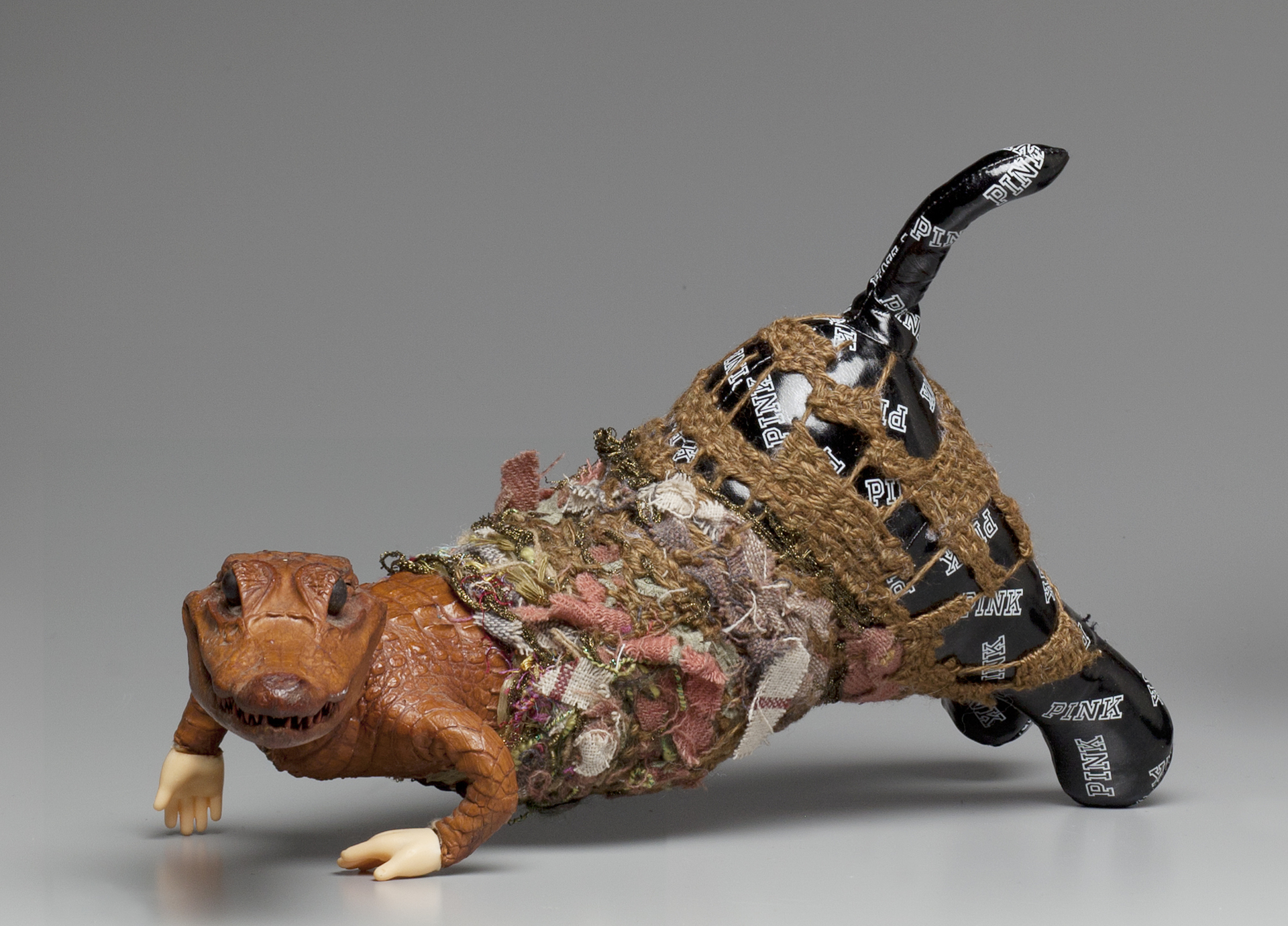This sculpture is an intricate composite of various materials, merging taxidermy, fabric, and ceramic elements. The creation features an alligator's head, its brown hide meticulously preserved, staring directly ahead with an unsettling lifelike gaze. In place of its original claws, the alligator's forelimbs are replaced with tiny, human flesh-colored doll hands. The midsection of the figure is an eclectic mix of fabric scraps and materials, pieced together to form a textured body. The sculpture transitions into the glossy black ceramic hindquarters of a cat, adorned with the word “PINK” repeatedly printed in white. A protruding black tail completes this bizarre yet captivating piece, seamlessly blending the natural and the artificial.